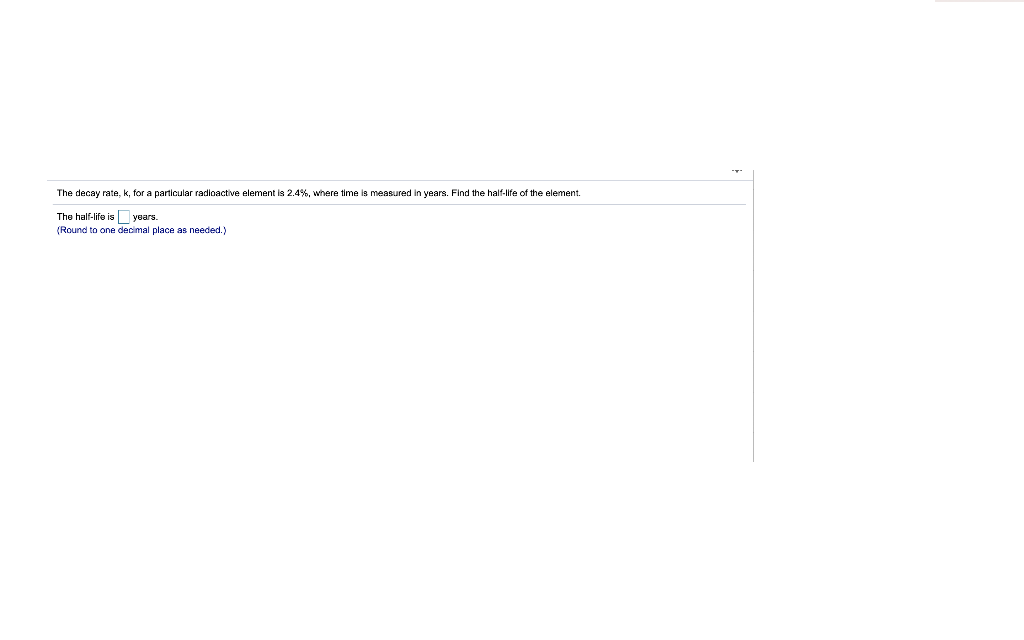The image presents a simple layout resembling a physics quiz question, possibly sourced from a web page. The design features a thick gray horizontal line extending across the top of the image. At the far right end of this line, the lower portion of a logo is visible, suggesting the upper part of the screen is not shown. Below this, a second, narrower gray horizontal line creates a wide rectangular box with the first line. A long gray vertical line extends downward from the bottom right of the box, marking the right-hand boundary.

Inside this rectangular box, the text reads: "The decay rate, K, for a particular radioactive element is 2.4%, where time is measured in years. Find the half-life of the element." This is followed by instructions indicating that the detailed work should be completed separately, as only the final answer is to be input into a provided box. The text prompts, "The half-life is," followed by a blank square to enter the number, with "years" immediately after it. Below this, in blue parentheses, it notes, "round to one decimal place as needed."

The format and content suggest it is part of a physics quiz, suitable for either high school or college courses, or potentially a standardized test.